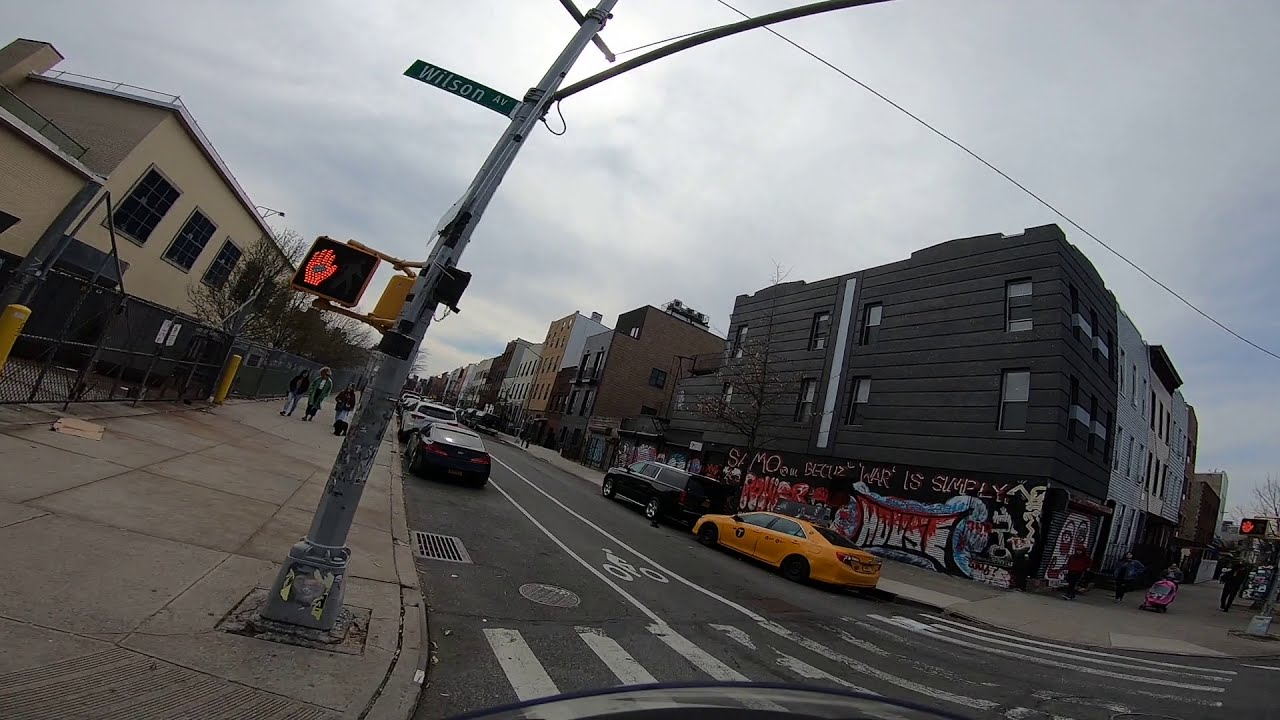The image captures a street view of an urban area on a cloudy day, with a road running diagonally from the bottom right corner to the top left. At the bottom right, a pedestrian crosswalk is marked by white lines. Moving towards the center of the road, a bicycle lane is indicated with two white lines and a painted figure on a bike. Rectangular buildings flank both sides of the street, featuring a variety of colors including black, brown, tan, white, dark gray, blue, and adorned with various graffiti, particularly on the right side. The building closest to the right features alternating dark gray, blue, and white sections. There's a yellow car parked behind a black SUV near this building. The road is essentially centered within the image, which is slightly tilted about 30 degrees clockwise, giving the impression that everything is leaning to the right. A street sign at the crosswalk displays a hand signaling 'stop.' The sidewalk on the left side shows a few buildings and a gate, while people stroll on the sidewalks on both sides of the road. In the distance, additional parked cars, including a black and a white one, fade away from view. This setting is denoted as Wilson Avenue, with its sign visible amidst a sky filled with clouds.